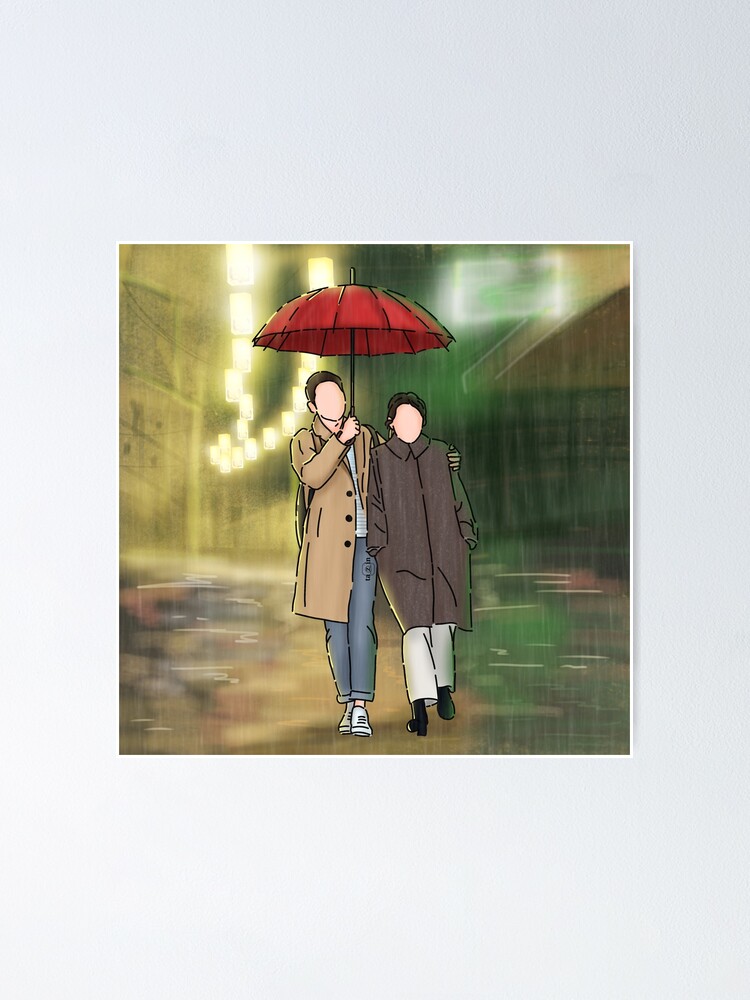In a blurred, rainy backdrop that suggests an overcast sky, the cartoon-like image depicts a vague, faceless scene. At the forefront are two individuals—perhaps a man and woman—both with smooth, featureless faces. The woman, with black hair, is dressed in a long, dark brown trench coat, white pants, black socks, and black shoes. Beside her is a slightly taller figure, possibly male, wearing a light brown trench coat over blue jeans rolled at the cuffs, a blue shirt, and white shoes. He extends his left arm to embrace the woman, sheltering both under a vibrant red umbrella as the rain pours down. The background, though indistinct, hints at a park with perhaps little houses, emphasizing the downpour against an otherwise muted setting.